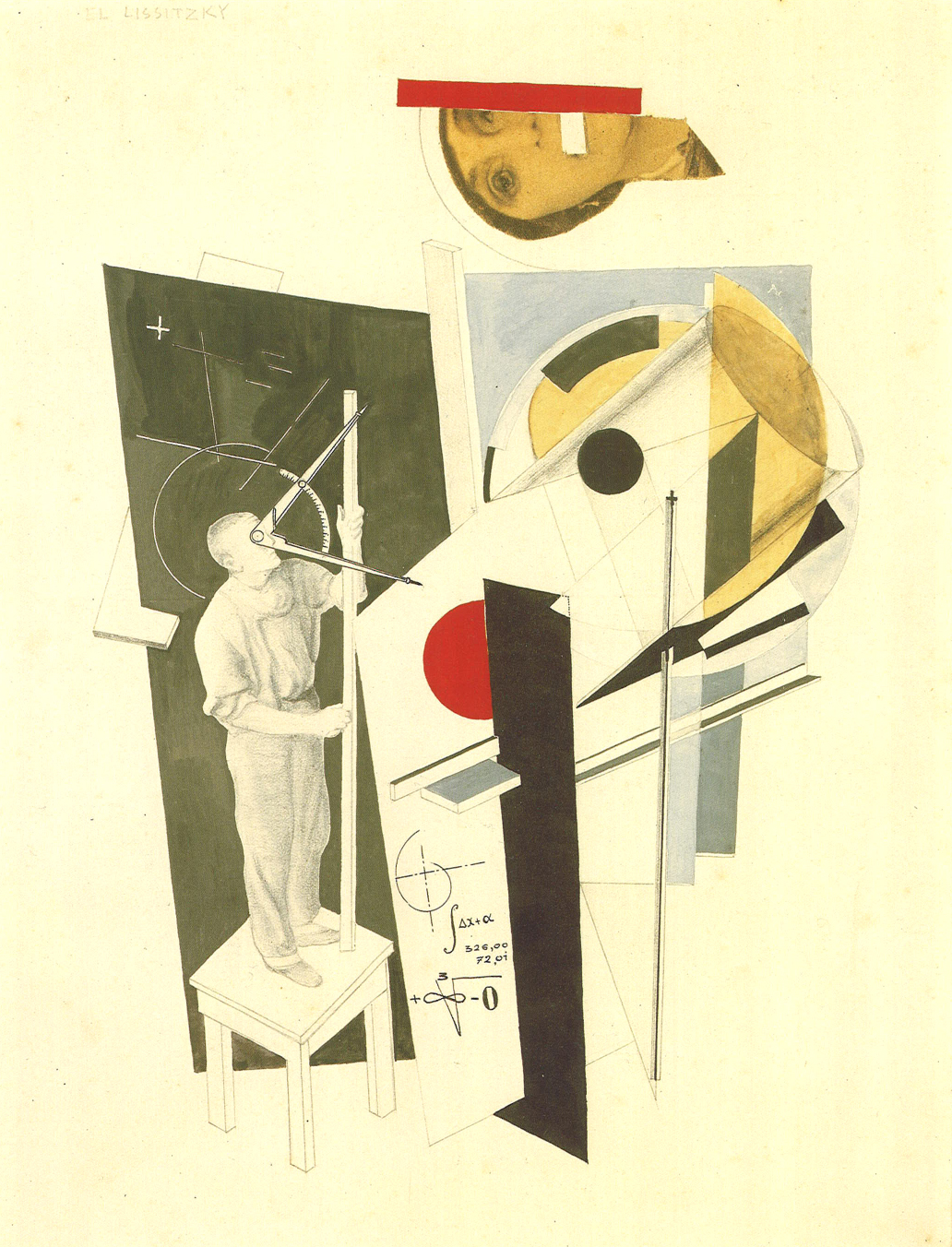The artwork in question is an abstract painting, likely executed on a yellowish aged paper or canvas, exhibiting elements that blend with pop art aesthetics. Dominated by black and white hues, the composition is accentuated with touches of yellow, red, gold, gray, and beige. Central to the piece is a male figure clad in a loose shirt with sleeves reaching his elbows and long pants, standing perched on a three-legged, possibly four-legged, table. He holds a tall meter stick that extends beyond his head. His face is obscured by an angle projector, embodying a mathematical theme, with a nearby chalkboard enhancing this scholarly atmosphere.

Surrounding the man are various geometrical shapes—squares, circles, half-circles, and parallelograms—in an array of colors including blue, black, white, yellow, and red. At his feet lies a math equation that involves the numbers 326, symbols like plus, minus, and zero, signifying computational processes.

In the upper region of the composition, a woman’s head appears laid sideways. Her face is largely masked by a bold red stripe, and her mouth is replaced by a white rectangle, presenting a motif of silence or censorship. The background bears faint, almost spectral, text including the name “Lissitzky,” an apparent nod to artist El Lissitzky. The entire scene is enshrouded in an environment that evokes deep contemplation of mathematical, artistic, and possibly societal themes, all rendered in an expressive and abstract manner.